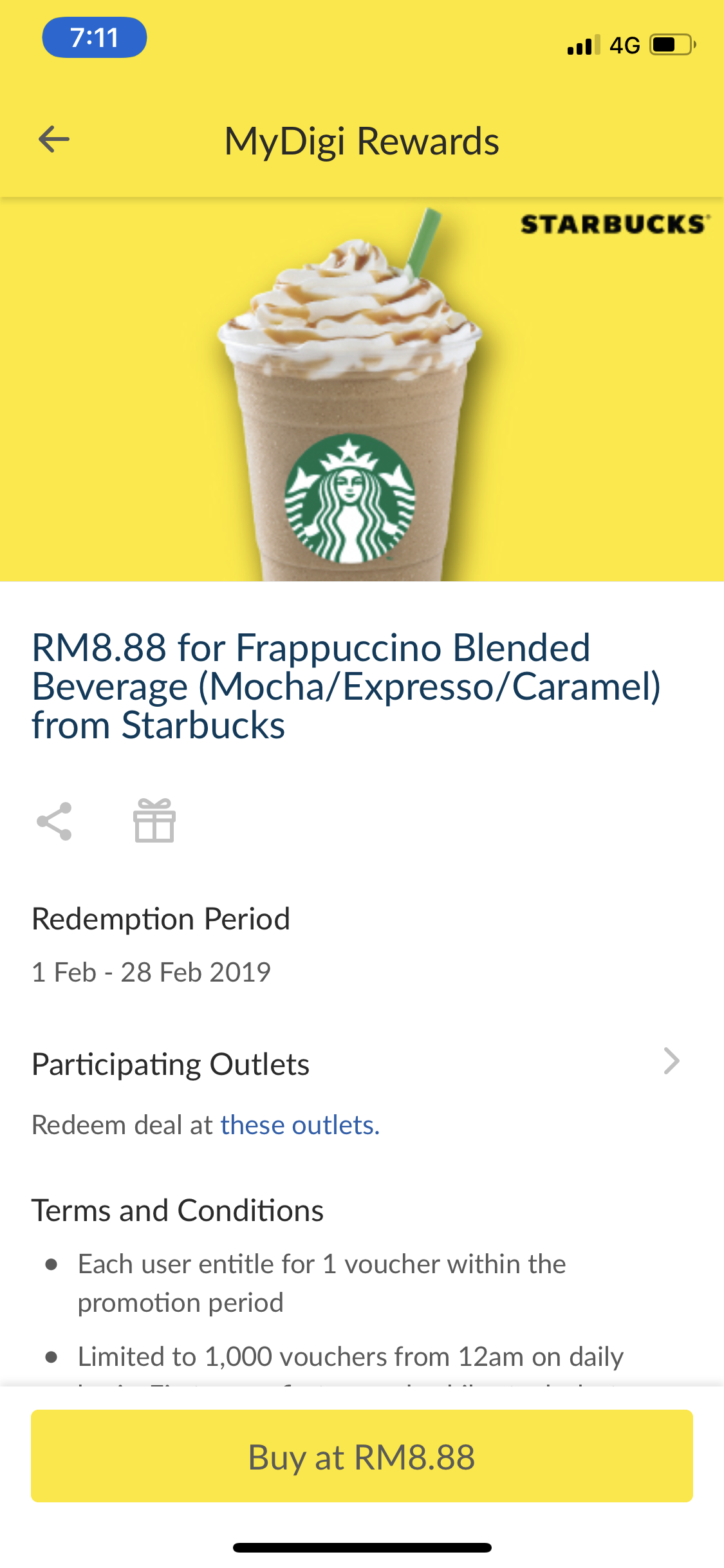Screenshot from a phone featuring a promotional offer for Starbucks:

At the top of the screenshot, the background is yellow. In the top left corner, the time is displayed as 7:11, and to the right, the battery level is shown to be slightly above 50%. Below this, there is a left-pointing arrow followed by the text "My DigiTree Rewards" and a faint green line. To the right of this line, in black letters, it says "Starbucks."

Centrally in the yellow section, there is an image of a Starbucks drink, likely a Frappuccino. The drink appears to be frozen with whipped cream and caramel sauce on top, finished with a green straw.

Below the image, the text reads:

"RM 8.8 for Frappuccino (blended beverage, mocha, espresso, caramel). Redemption period: 1 February - 28 February 2019. Participating outlets: redeemable at these outlets."

Further down, the terms and conditions are provided: 

"Each user is entitled to one voucher within the promotional period, limited to 1,000 vouchers daily starting from 12am."

At the bottom of the screen, the background turns yellow again with the offer "Buy at RM 8.88" followed by a black line at the very bottom.